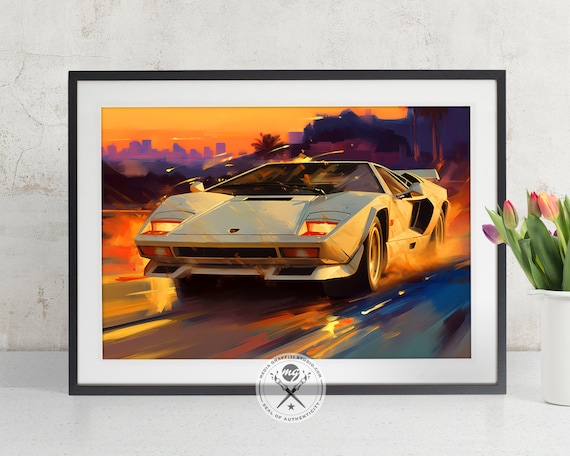The image is a square, colorful painting of a white Lamborghini Countach, showcased in a black wooden frame with a white border. The sleek, angular sports car, reminiscent of the fast, iconic 1980s design, is depicted driving on wet pavement, causing splashes of water around its tires. Its headlights are on, illuminating the rain-streaked road which features vibrant streaks of blue, orange, and purple. The backdrop reveals a cityscape with skyscrapers and an orange-tinted sunset sky turning into a purple silhouette. Positioned in the lower left corner of the image, on a white countertop against a minimalist white wall, is a white vase containing green leaves and tulips. A circular watermark with unreadable black text is located at the bottom center of the image, adding a subtle detail to the overall composition.